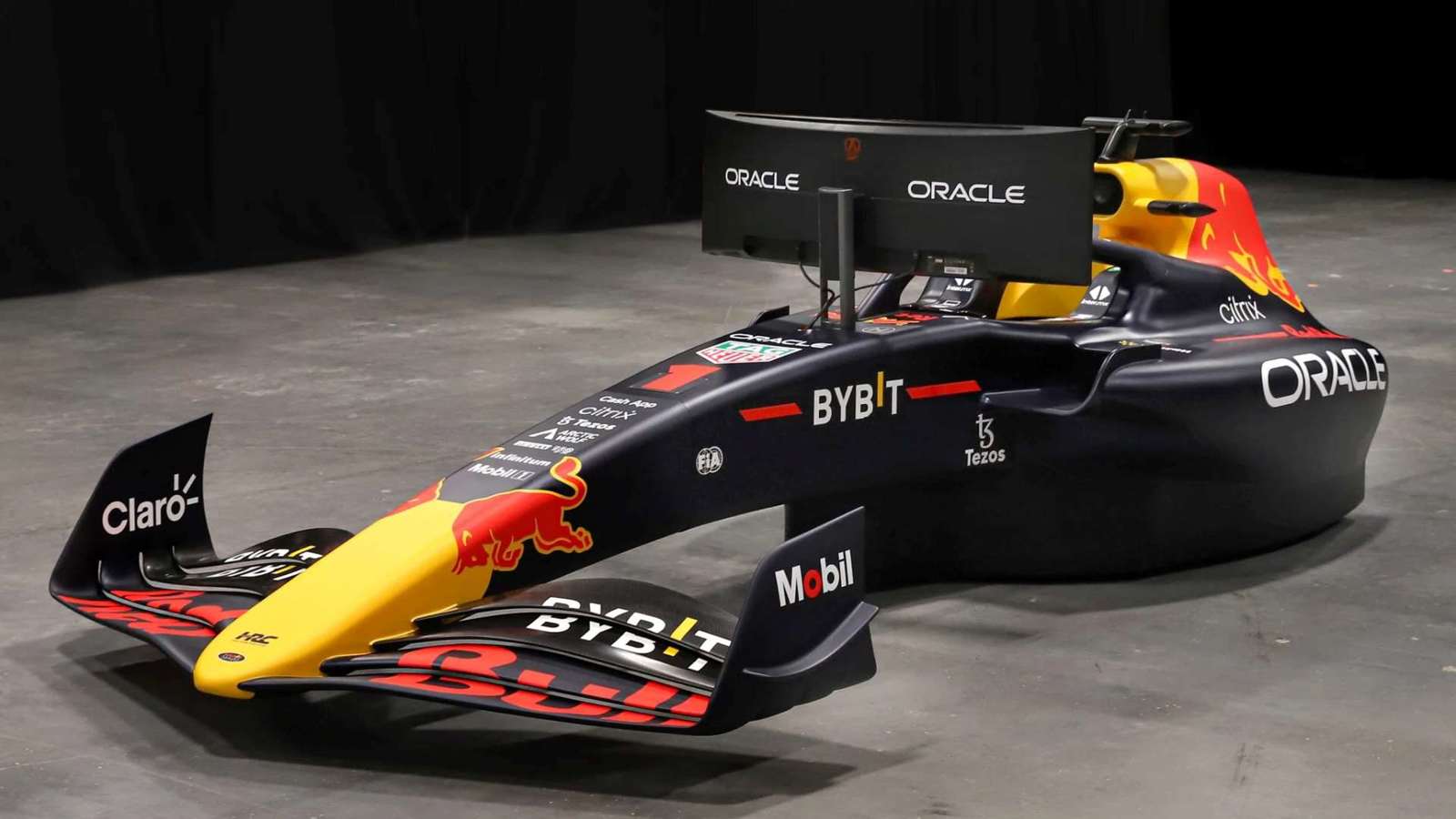This indoor photograph captures a unique, futuristic vehicle, potentially a concept race car or boat, positioned on a gray concrete floor against a black wall backdrop. The vehicle boasts a sleek, elongated black body accented with vibrant yellow and red markings. The tip of the nose is yellow, adorned with two red bull logos facing each other, and is situated in the lower left-hand corner of the image. At the front, two upturned black wings feature red and white sponsor labels reading "Claro" and "Mobile." The vehicle is heavily branded, with "Oracle" prominently displayed in large white letters on the sides and the back. The rear of the vehicle, which starts in the upper right-hand corner, showcases a cockpit area with a wide, curved monitor, also labeled "Oracle" on the back. Additional sponsors, including "Bybit," "Mobil," and "Claro," are scattered across the body of the vehicle. The combination of its sleek, aerodynamic design and corporate branding suggests a high-tech simulator or concept model, blending elements of both automotive and nautical forms.